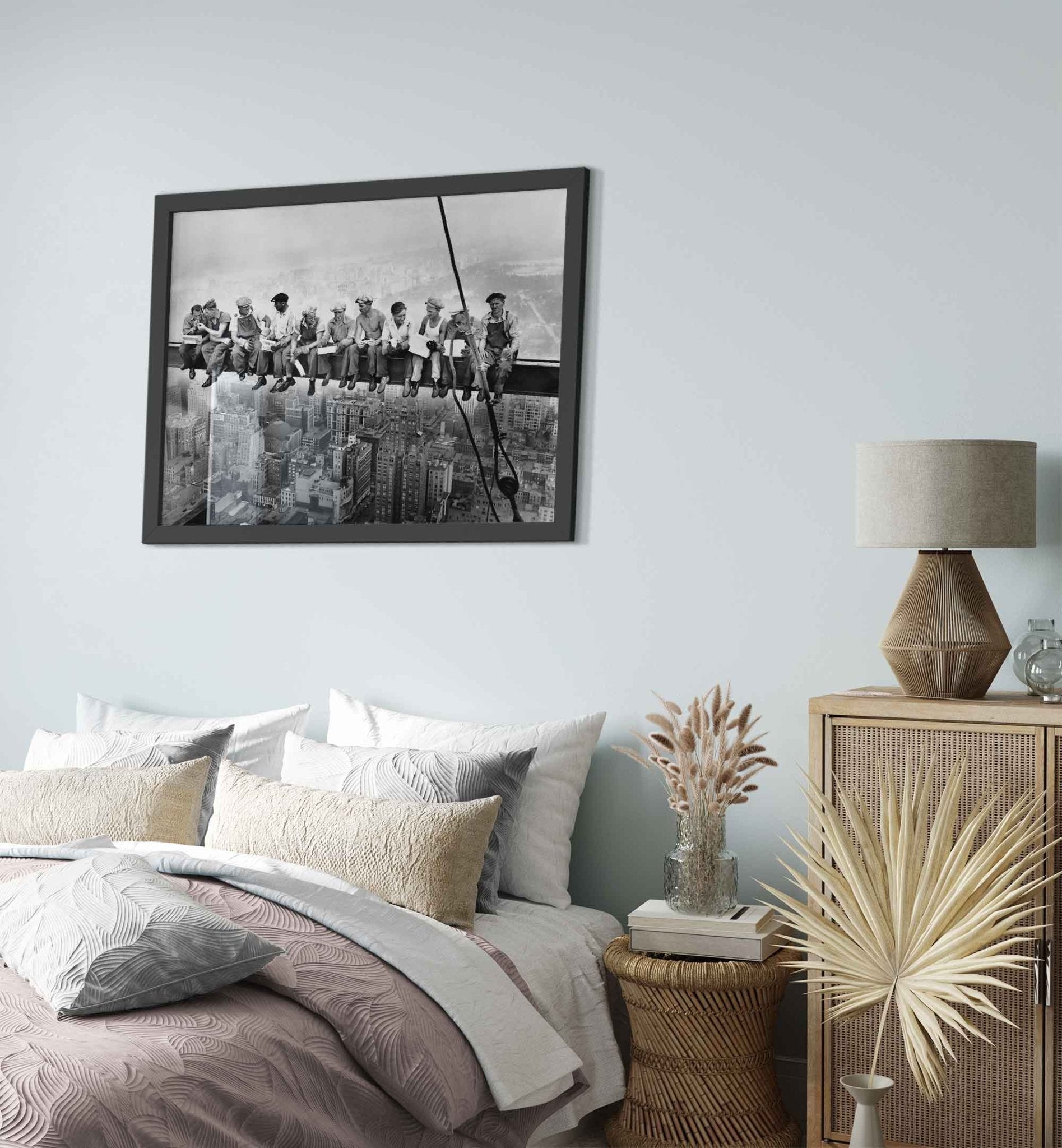In this image of a meticulously arranged bedroom, a bed sits prominently on the left side. The bed, adorned with a brown bedspread, features an array of seven pillows. The pillows are organized with two large white ones at the back, two smaller gray ones in front, followed by even smaller yellow ones, and an additional gray pillow lying on top. Above the bed, a black and white framed photograph hangs, depicting construction workers on a beam overlooking a vast cityscape.

Next to the bed, two nightstands flank with distinct setups. On one side, there is a wicker nightstand with a stack of two books and a floral arrangement on top. On the other side, a larger dresser supports a wooden lamp with a white or gray lampshade, complemented by a smaller glass vase. Additionally, there's another larger white vase with an intricate beige floral arrangement positioned directly on the floor in front of it. The wall behind the bed is painted a soothing light blue, contributing to the room's tranquil ambiance.